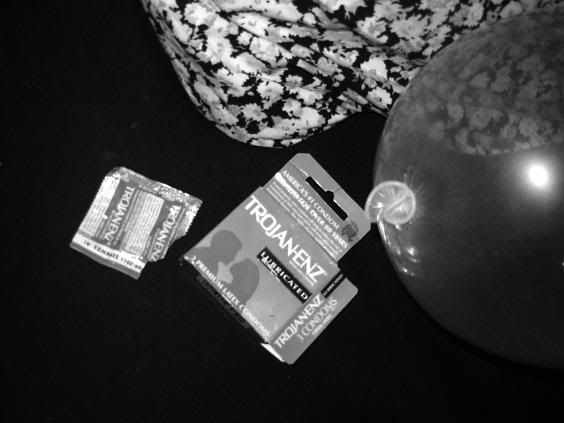This grayscale advertisement for Trojan ENZ lubricated condoms prominently features a centrally placed, open box of Trojan condoms against a black background. To the left of the box, an open Trojan condom wrapper is visible. At the top edge of the image, there's a hint of what appears to be a floral patterned blanket or sheet, suggesting the edge of a bed. On the right side, there seems to be an inflated condom or balloon, which has a shiny, transparent appearance. The entire image is overlaid with a watermark that includes a circular, swirly pattern labeled "photo bucket," and an opaque bar near the bottom reading "protect more of your memories for less."